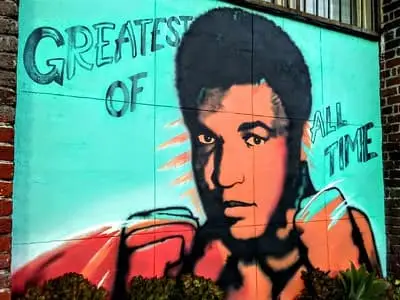This detailed descriptive caption brings together the key elements shared across the different descriptions, emphasizing the repeated details.

---

The image showcases a vibrant mural of Muhammad Ali, capturing his iconic status as the "greatest of all time." Painted on a brick wall in an urban setting, Ali is depicted in his younger days, standing in a classic boxer's pose with high afro hair, his fists raised in the air. The mural spans the entire wall, with a backdrop of aqua green. The phrase "greatest of all time" is prominently displayed, with "greatest of" positioned above his head and "all time" to the right. The letters are rendered in black. The mural features a rich color palette, including browns, blacks, oranges, and greens, with a noticeable reddish hue in the lower left corner. Additionally, there are some plants in front of the mural, enhancing the outdoor ambiance. The setting is well-lit with natural light, making the vibrant details of the mural and the surrounding environment clearly visible.